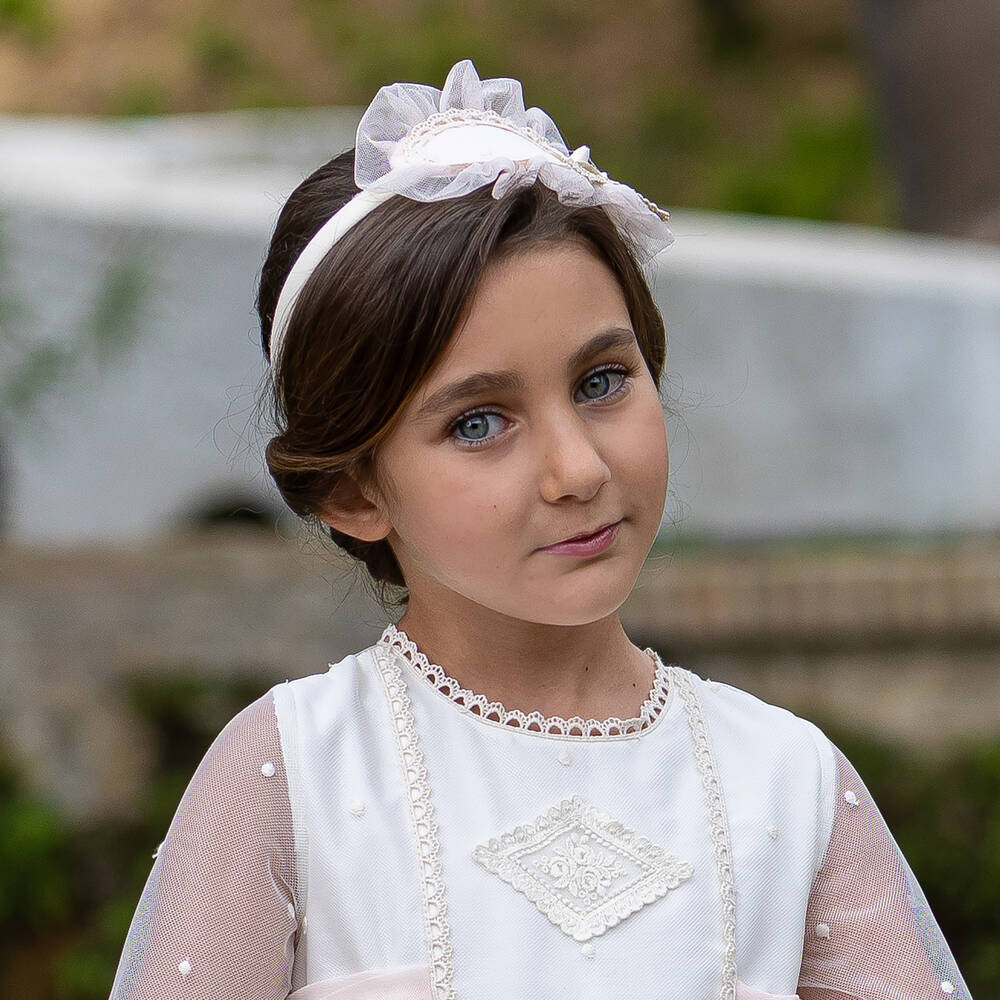The photograph captures a young girl, approximately eight to ten years old, standing outdoors with a blurred wooded area in the background. She is positioned in front of a large, light-colored concrete slab with some visible black on one side, and a wooden railing with green patches. The girl has medium-toned skin, pale blue-gray eyes, dark brown hair pulled back, and wears a white headband adorned with lace and frills. Her white dress is intricately detailed with scalloped lace around the collar, a diamond-shaped lace emblem on her chest, and sheer, mesh sleeves dotted with small, white pearls. The background, although out of focus, hints at a combination of cement walls and greenery, further enhancing the serene outdoor setting.